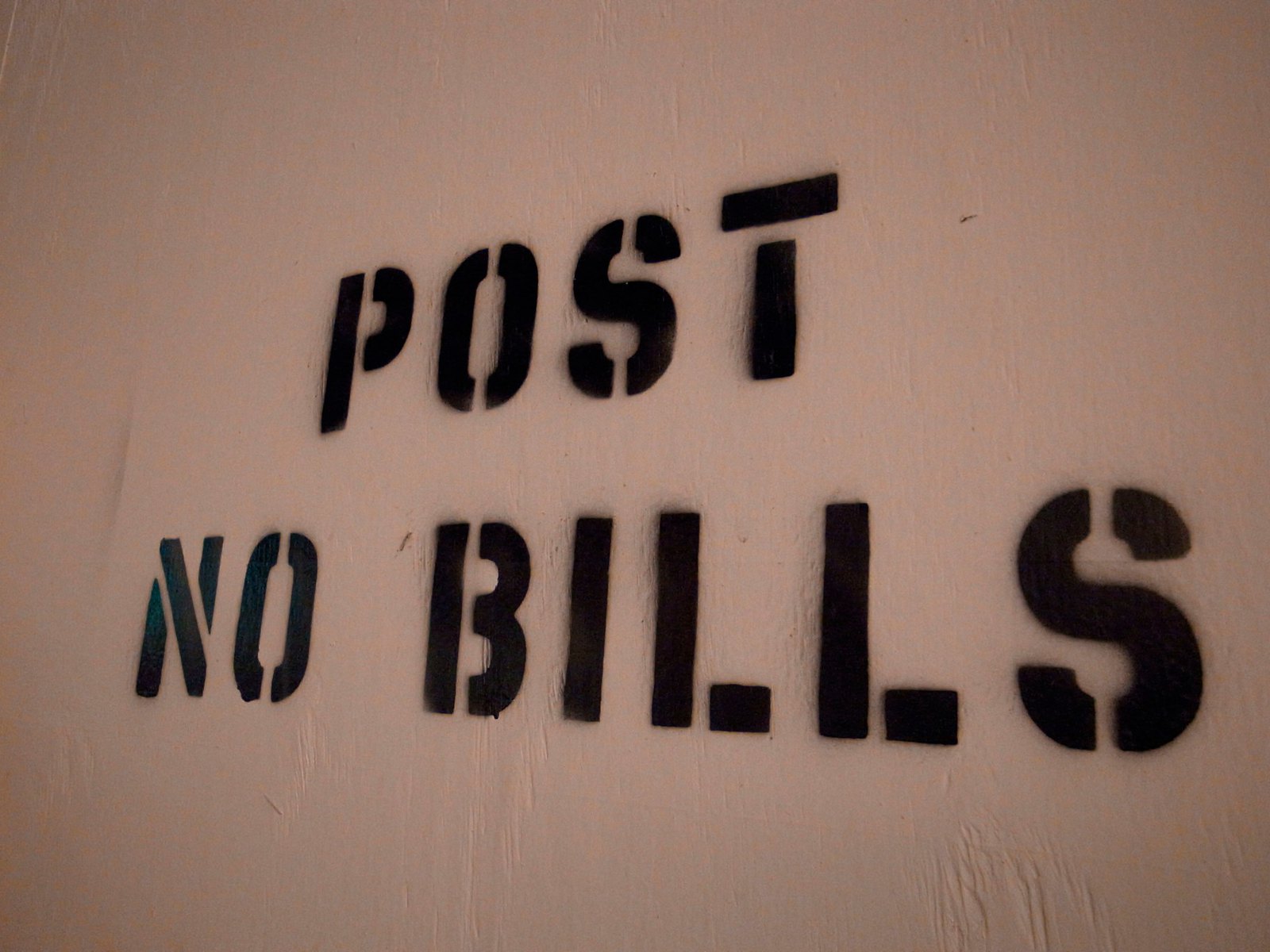The image depicts a rough and irregular wall, seemingly painted over in white, featuring a stenciled message in black spray paint that reads "Post No Bills." The stenciled lettering appears fragmented, with distinctive breaks in the letters due to the stencil design. For instance, the "P" in "Post" comprises a vertical bar and a detached curved segment, the "O" appears split in two, and the "S" is divided into three separate parts. This creates a retro, 80s-style aesthetic reminiscent of signs seen around New York City. The photograph captures the sign at an angle, slightly off to the right, causing the text to appear smaller on the left side. The background and specific location are indeterminate due to the close-up nature of the photo.